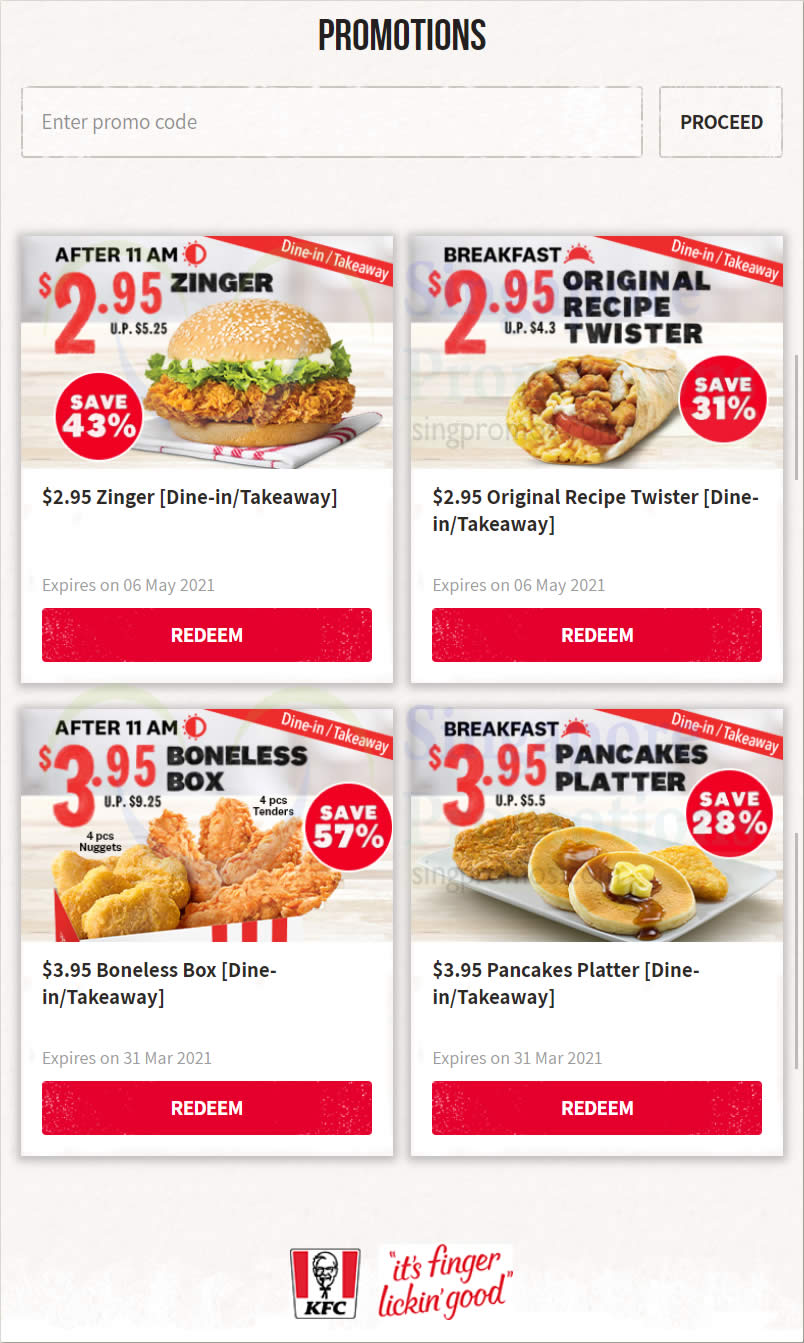The image features a light purple background with the title "Promotions" prominently displayed at the top. Below this, there is a field labeled "Enter Promo Code" followed by a "Proceed" button.

The image is divided into four promotional boxes, each containing specific details:

1. The first box promotes a "Zinger" deal available after 11 a.m. for $2.95, highlighted in red. There is a banner across this box indicating "Drive-In, Take-Away" with a 43% savings. It includes a red "Redeem" button at the bottom.

2. The second box advertises a "Original Recipe Twister" available for breakfast, priced at $2.95. A red flag denotes "Drive-In, Take-Away" with a 31% discount. This box also features a red "Redeem" button.

3. The third box showcases a "Boneless Box" available after 11 a.m. for $3.95, with a substantial 57% saving indicated by a banner. It is marked for "Drive-In, Take-Away" and includes a red "Redeem" button.

4. The fourth box highlights a "Pancake Platter" breakfast deal for $3.95, saving 28%. This box is also tagged with "Drive-In, Take-Away" and features a red "Redeem" button.

At the bottom of the image, the light purple background continues, featuring the KFC insignia—a red and white box with Colonel Sanders’ face and the text "KFC" alongside the slogan "It's finger-lickin' good" in red.